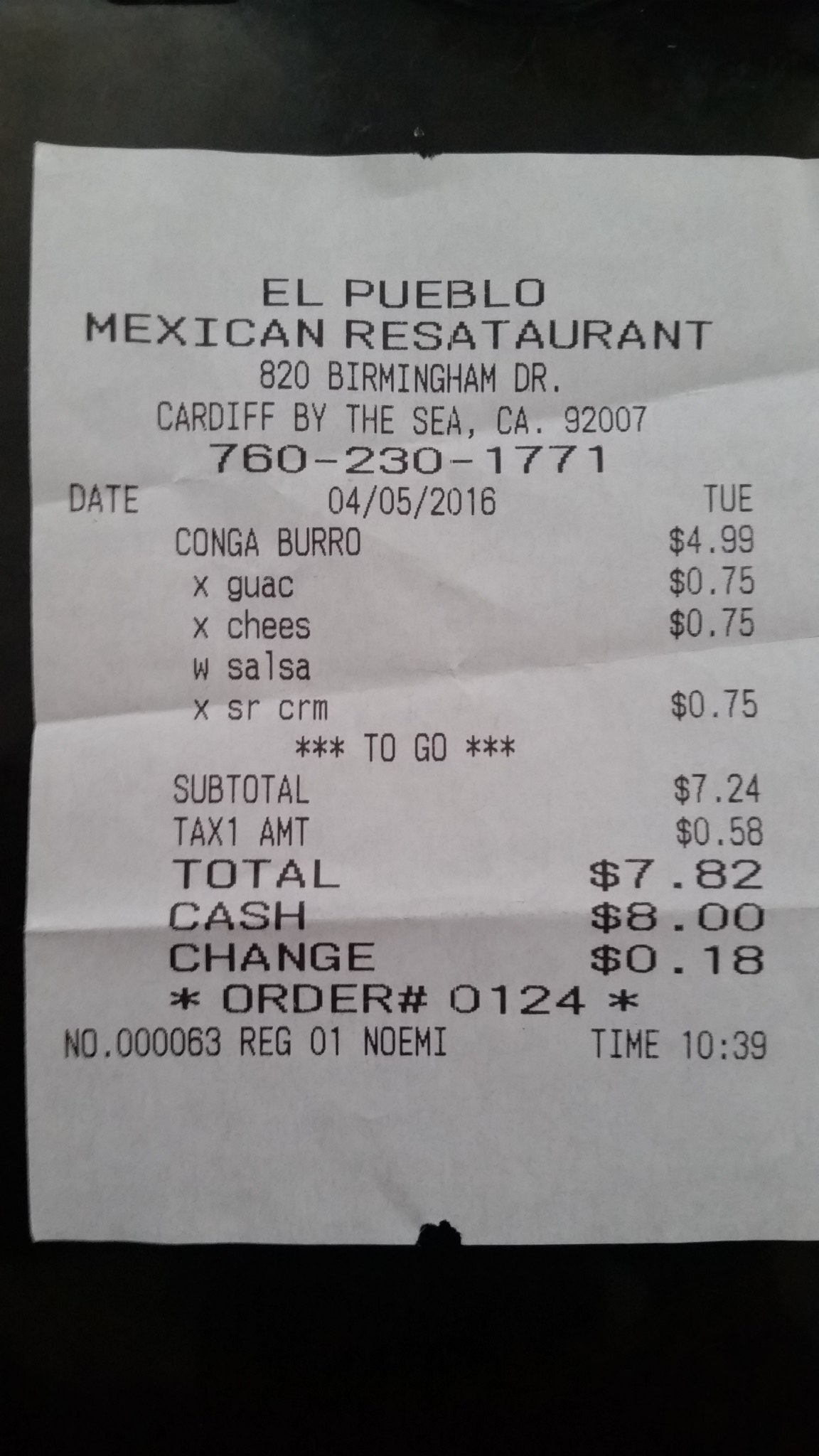This image features a small, white receipt photographed against a reflective black surface. The receipt is from El Pueblo Mexican Restaurant, located at 820 Birmingham Drive, Cardiff by the Sea, California, 92007. The restaurant's phone number, 760-230-1771, is also prominently displayed. Dated April 5th, 2016 (a Tuesday), the receipt details each item ordered, including a "Conga Burro" priced at $4.99, with additional charges for guacamole, cheese, salsa, and sour cream at $0.75 each. The subtotal is $7.24, with a tax amount of $0.58, bringing the total to $7.82. The customer paid in cash ($8.00) and received $0.18 in change. Additional details at the bottom of the receipt include the order number (0124), the time of purchase (10:39), and the cashier's name (Naomi).